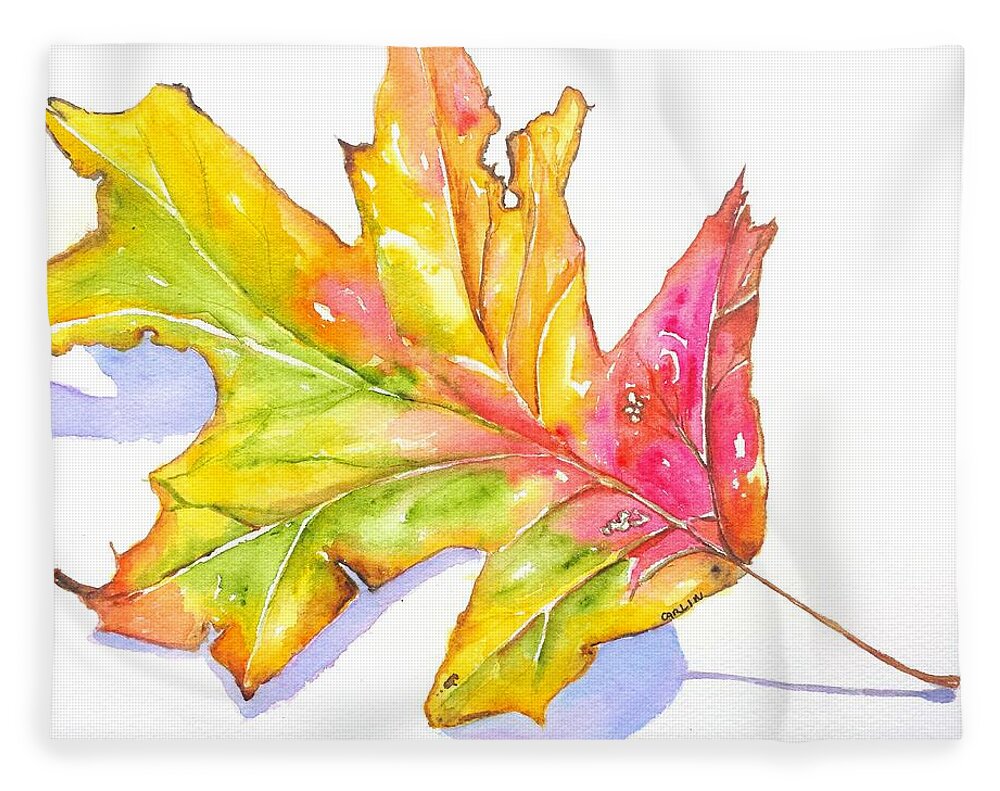The artistic piece depicts a vibrant, watercolor maple leaf set diagonally against a white background with a subtle, light gray checkered pattern. The leaf shows a dynamic array of colors: the upper portion features hues of red, yellow, and pink while the lower portion transitions into light green, yellow, and orange. The stem is a light brown, extending towards the lower right corner. A light purple reflection of the leaf and stem adds depth to the image. The overall composition is reminiscent of fine art, known for its pastel and prominent edge colors such as orange and gold. The veins within the leaf blend white and greenish tones, with the stem displaying a reddish-brown hue. Shadows beneath the leaf enhance its dimensionality. The creator's signature, "Galen," is inscribed in black at the bottom left corner of the image.